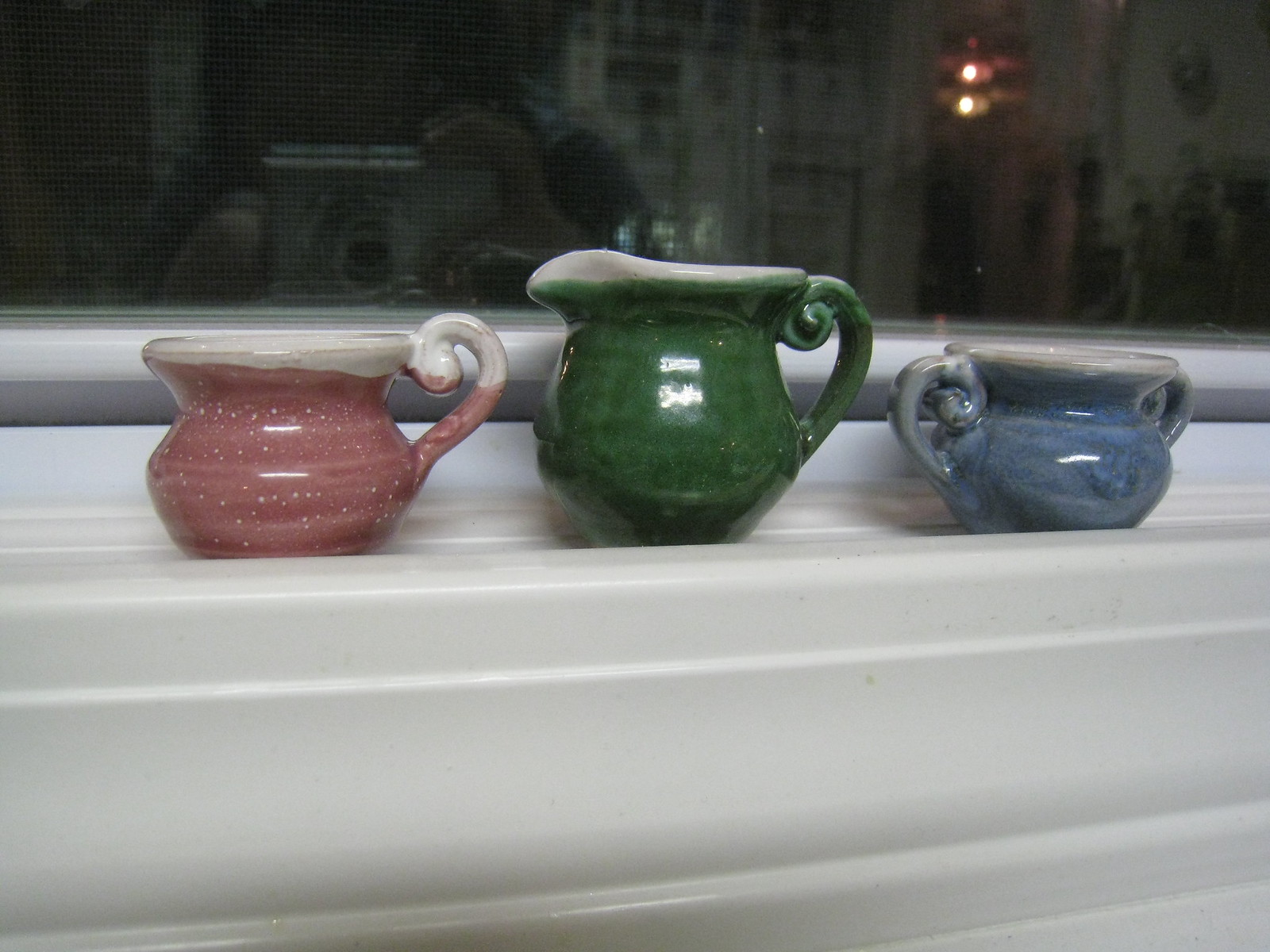In this nighttime photograph, taken from inside a well-lit room, three ceramic pots are neatly lined up on a windowsill, creating an intriguing still life. In the background, a window reflects the dimly lit exterior, mirroring everything behind the camera. Within this reflection, the silhouette of the photographer, clad in a blue shirt and holding a silver digital camera, is faintly visible. The pots are of varying sizes and colors, each with a handle and a spout, indicating they are likely used for pouring beverages. The pot on the left, a medium-sized vessel, is a pinkish-red hue with speckled details. The middle pot stands tallest in a dark green shade, noticeably more prominent than its counterparts. On the right, the smallest pot is a blue color, unique with handles on both ends and a more intricate jug-like shape. All the pots are ceramic, glazed with a sheen that catches the light, and their interiors are a crisp white. The arrangement, combined with the reflective window, creates a visually layered and captivating image.